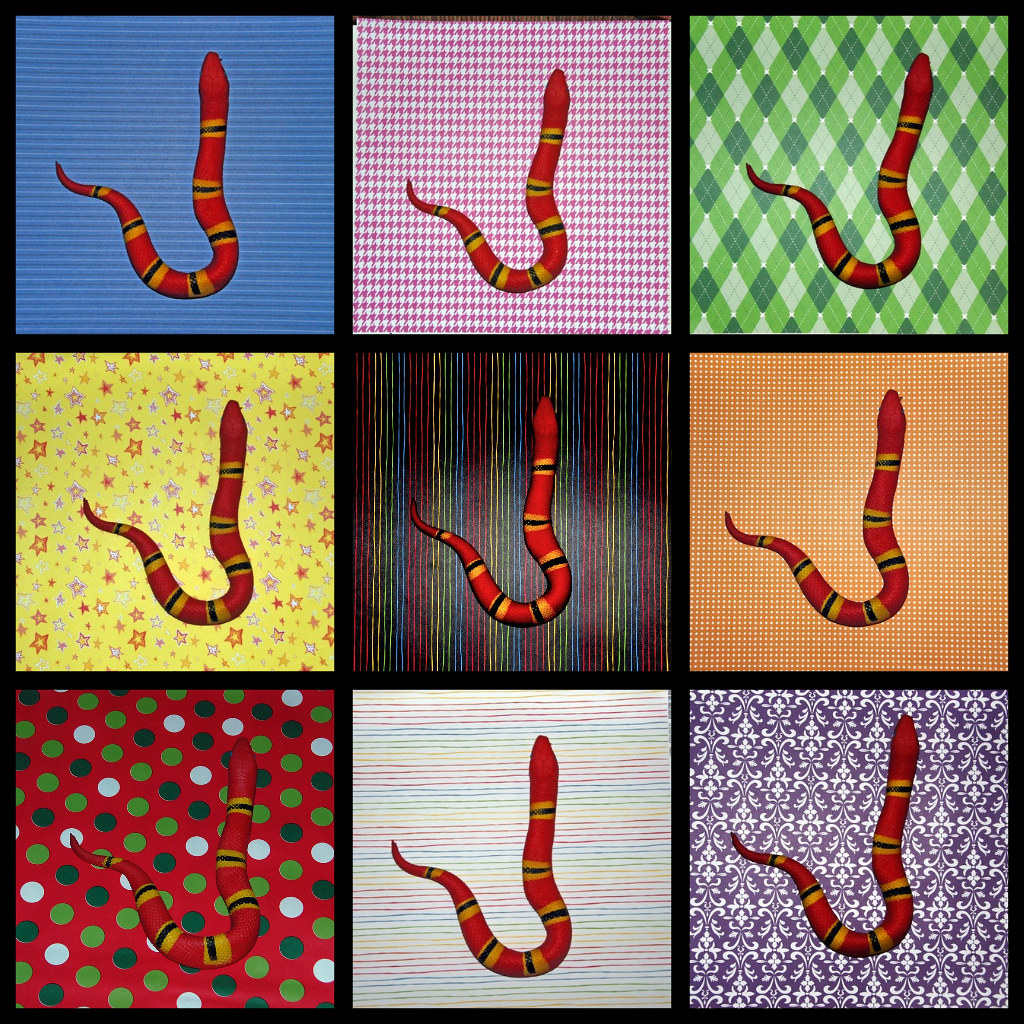The image is a digitally created piece of artwork featuring an artistic representation of a snake, possibly a coral snake or corn snake, displayed in a 3x3 grid of square tiles, totaling nine squares. Each tile exhibits the same uncoiled red snake adorned with alternating yellow and black bands, consistently positioned in a hook-like shape across all tiles. The backgrounds of each square differ uniquely:

- The top left square has a royal blue background with subtle stripes.
- The top middle square features a red and white gingham pattern.
- The top right square showcases a diamond pattern in shades of light green, dark green, and white.
- The middle left square has a yellow background adorned with red and white stars.
- The center square in the middle row presents a background with rainbow-colored stripes.
- The middle right square displays an orange and white checkered pattern.
- The bottom left square is red with white, dark green, and light green polka dots.
- The bottom middle square contains horizontal pastel stripes in yellow, blue, and pink.
- The bottom right square features a purple background with intricate white geometric scroll designs.

This detailed repetition of the snake against varied, vibrant backgrounds creates a visually dynamic and colorful artwork.